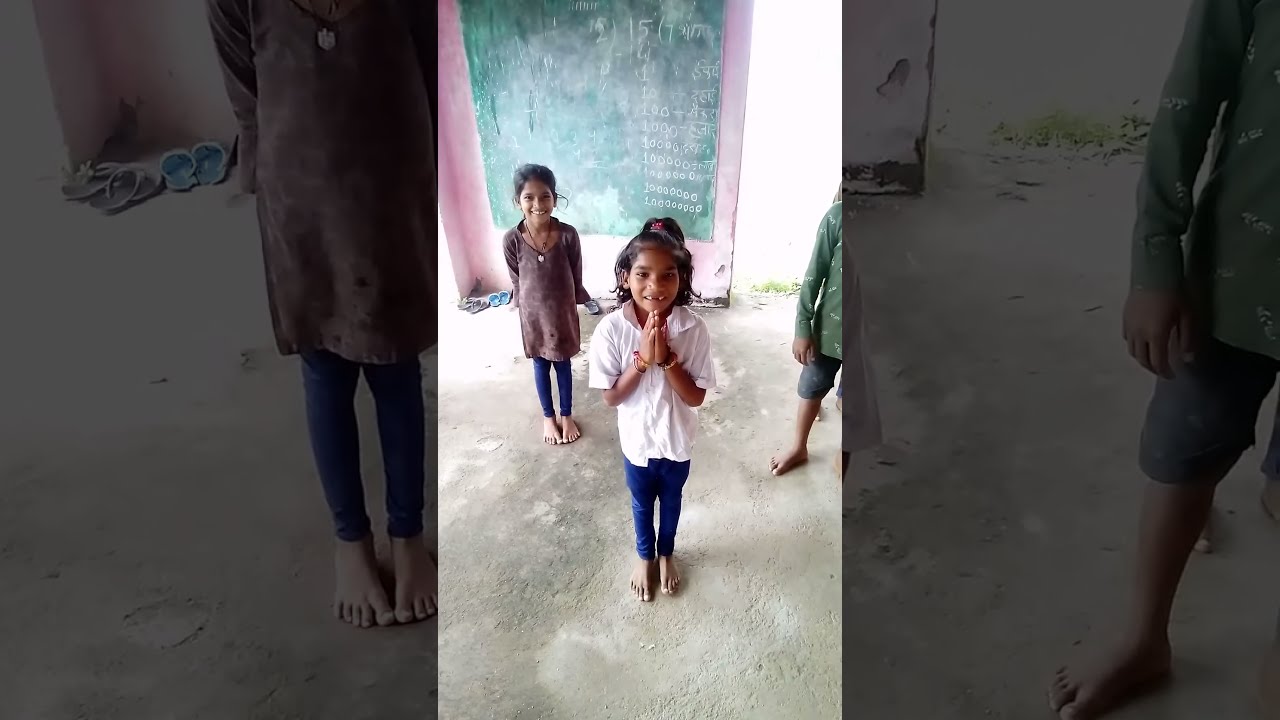The photograph features three young children, likely from India or a similar region, standing barefoot on a dirt or stone floor within a structure that appears dilapidated. The building has a roof, casting shadows, while sunlight seeps in, suggesting an indoor setting with external light. Behind the children is a green chalkboard mounted on a pink wall, displaying chalk-written numbers, primarily ones and zeros. The children, who seem around five or six years old, are dressed in somewhat soiled and worn clothing: the central figure, a girl, sports a light pink short-sleeved shirt; another girl behind her wears a red shirt; and the boy in the back is clad in a green shirt and blue shorts. The scene includes scattered sandals or shoes in the background, adding to the impression of poverty. Despite their surroundings, the children appear content and happy, depicting resilience amidst challenging conditions.